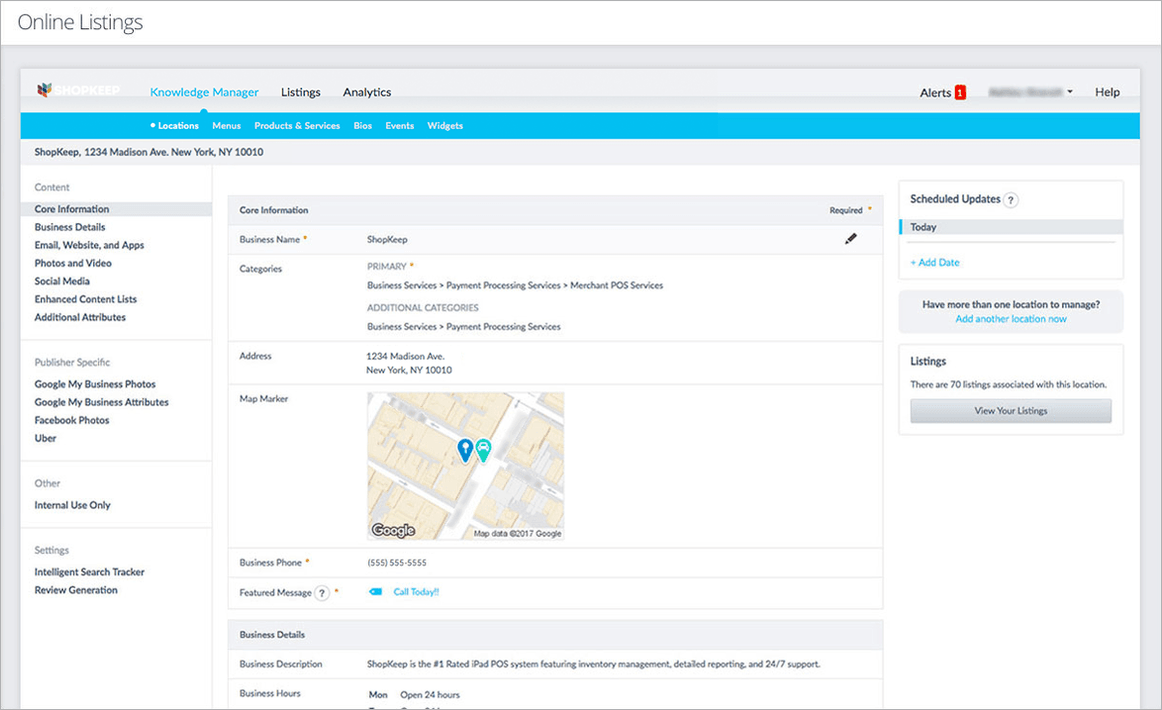This screenshot features a white background and starts with the heading "Online Listings" in grey letters at the top. Below this, there is a grey-bordered rectangle with a white interior. Within this section, the following elements are displayed:

1. **Tabs and Navigation**:
   - The blue tab labeled "Knowledge Manager" is open, with "Listings" and "Analytics" as additional headings in blue text. 
   - A blue banner below these tabs lists further headings in white text: "Locations," "Menus," "Products and Services," "Bios," "Events," and "Widgets."

2. **Business Information**:
   - In black letters, it reads: "Shop Keep, 1234 Madison Avenue, New York, New York, 10010."
   - On the left side, headings include "Content," "Publisher Specific," "Other," and "Settings," each with subheadings beneath.

3. **Main Content Area**:
   - A central rectangle displays core information:
       - **Business Name**: Shop Keep
       - **Categories**: Primary - Business Service; Payment Processing Service; Merchant POS Service
       - **Additional Categories**: Business Services; Payment Processing Services
       - **Address**: 1234 Madison Avenue, New York, New York
       - **Map Marker**: A map image featuring a teal-colored pinpoint indicating the location, with the word "Google" marking it as a Google Map snapshot.
       - **Business Phone Number**: 555-555-5555
       - **Feature Message**: Accompanied by a price tag icon, it reads "Call today."

4. **Business Details**:
   - **Business Description**: "Shop Keep is the number one rated iPad POS system, featuring inventory management, detailed reporting, and 24-7 support."
   - **Business Hours**: Monday, open 24 hours.